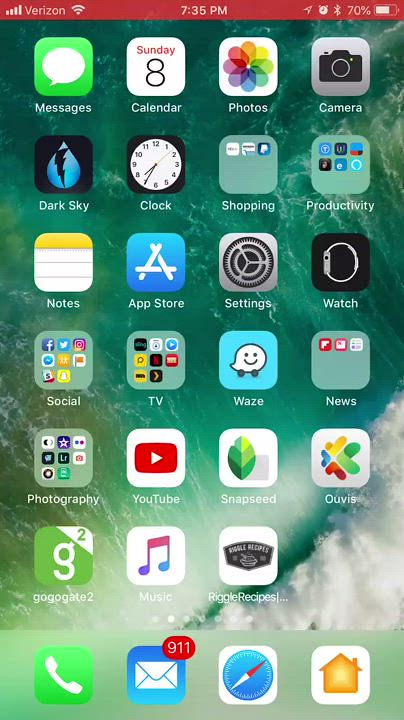The image captures a snapshot of a phone's home screen, showcasing a detailed view of the various app icons arranged neatly across the screen. The top left panel features icons for Messages, Calendar (displaying "Sunday 8th"), Photos, Camera (represented by a camera icon), Dark Sky, Clock, Shopping, and Productivity Notes. Moving downwards, you can see apps such as the App Store, Settings, Watch, Social, TV, Waze, News, Photography, YouTube, Snapseed, Populist, Music, and Rich Recipes, each accompanied by its unique icon indicative of its function.

Prominently, the background of the home screen features a vibrant and dynamic image of moving water, likely from an ocean or sea. The water exhibits a captivating blend of green and bluish hues, and appears to be splashing white foam against a surface located at the bottom-right corner.

At the bottom of the home screen, four larger icons are easily noticeable: one for Phone, one for Email, one for Web Browsing, and the Home Button.

At the top of the screen, the status bar displays several crucial indicators: on the left side, "Verizon" along with the Wi-Fi signal strength; in the center, the current time "7:35 PM"; and to the top right corner, various icons including the battery symbol, providing a comprehensive view of the phone's status.